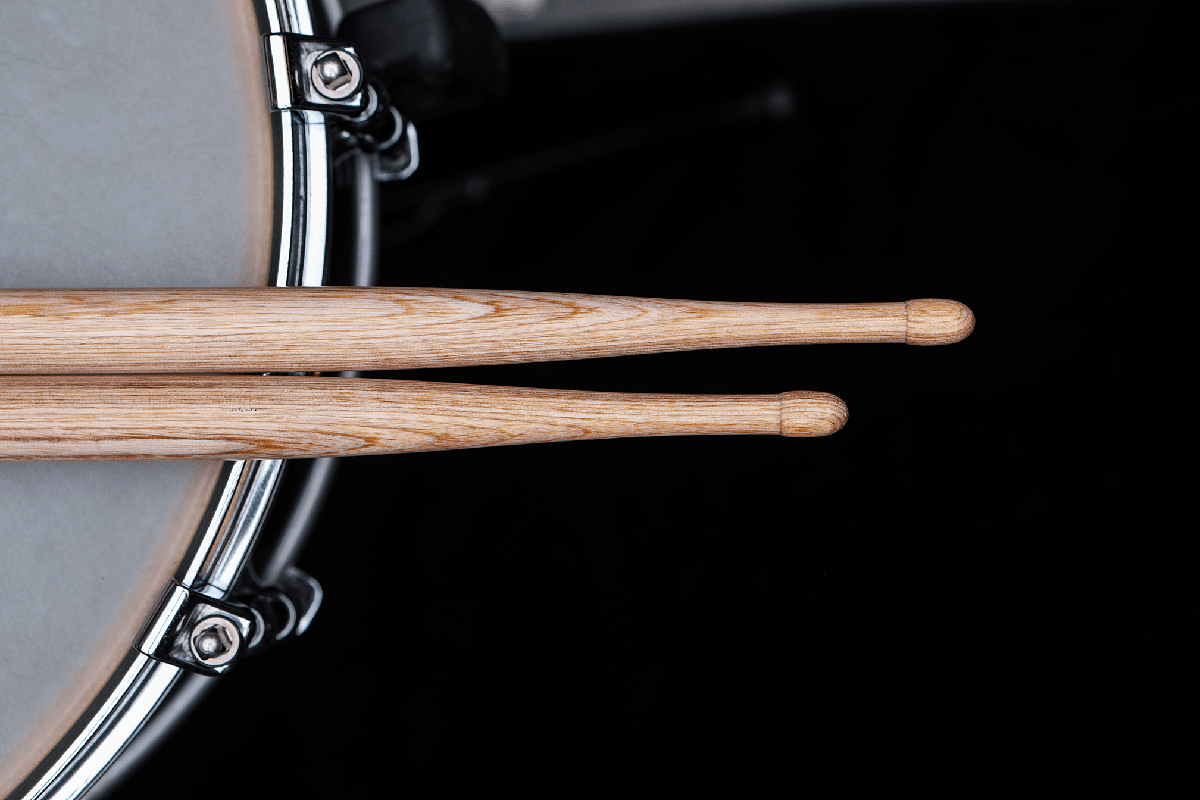The image is a professional close-up shot taken from above, showcasing the edge of a drum adorned with silver metal detailing. On the drum's light-colored surface, two light-colored wooden drumsticks, possibly made of pine, are positioned slightly hanging off its edge. The drumsticks, with clearly visible wood grain, lie across the drum, with their heads extending towards the right side of the picture. Only a small portion of the drum, specifically the bottom left segment, is visible in the image. The majority of the background is pitch black, likely due to the camera's flash, creating an almost empty void-like appearance. At the top of the image, a faint hint of what could be the rest of the drum kit is visible but remains out of focus. The image contains no text.